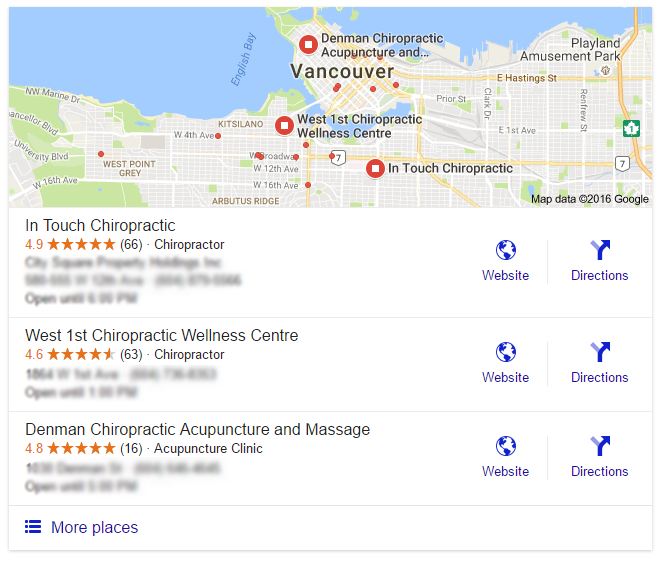This image features a detailed map of Vancouver, prominently displaying "Vancouver" in black letters at its center. Above this central label, the map highlights "Denman Chiropractic Acupuncture End." The layout suggests it is the result of a search query rather than an active search interface, as there is no visible search bar. 

The map is dotted with red circles containing white boxes, signifying the locations of chiropractic offices within Vancouver. Key landmarks such as English Bay are visible, providing geographic context. Below the map, a list of chiropractic businesses appears, likely generated by the search.

The first listed business is InTouch Chiropractic, boasting a five-star rating along with available website links and navigation directions. Following is West First Chiropractic Wellness Center, also featuring a website link and directions. Lastly, Denman Chiropractic Acupuncture and Massage is listed with similar detailed information. Additional operational details such as hours, addresses, and phone numbers are obscured, appearing grayed out.

Beneath these listings, there is an option to view more places via a clickable menu, inviting further exploration of additional chiropractic services in the area.